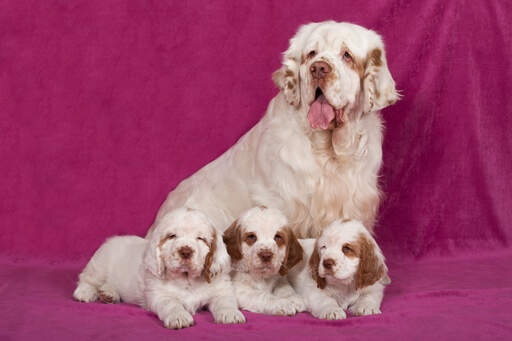The professionally-taken photograph captures a family of four dogs, prominently featuring a parent dog and its three adorable puppies. Set against a backdrop tinged with hues of dark purple and lava pink, the scene is meticulously arranged on what appears to be a studio floor rug, enhancing the image's polished aesthetic. Although the specific breeds are not identified, the dogs' fur is predominantly white with charming brown spots accentuating their faces. The parent dog stands watchfully behind, exuding a serene yet slightly energetic demeanor, while the three puppies, nestled comfortably in front, appear drowsy and content. The composition beautifully conveys a sense of familial warmth and professional artistry.